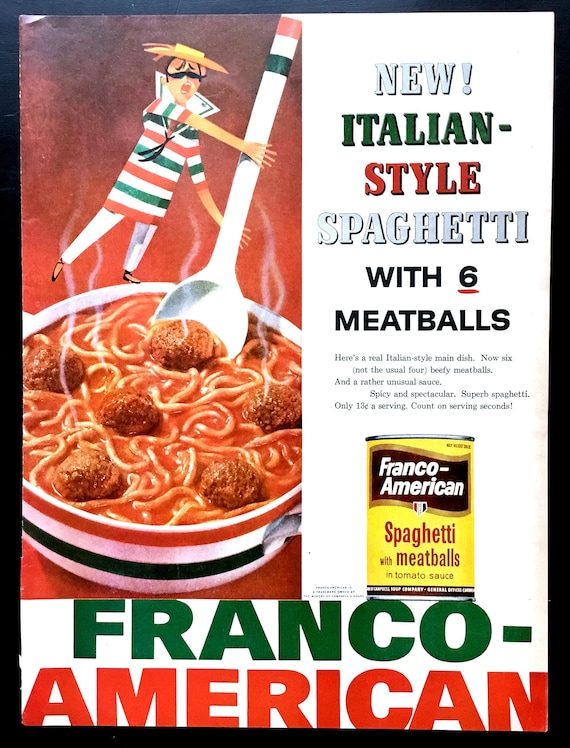The image is a vintage advertisement for Franco-American Spaghetti with Meatballs, likely from the 1950s or 60s, as suggested by its style and presentation. The ad features a cartoonish figure of an Italian man dressed in attire representing the Italian flag—orange, white, and green. The man wears a gondolier hat, white pants, and sports a large black mustache. He energetically stirs a steaming bowl of spaghetti and meatballs with a large spoon that also carries the Italian colors. The background has a black border framing the entire ad, which appears to be a magazine print.

Bold text announces "New! Italian-style Spaghetti with Six Meatballs" in an eye-catching combination of white, green, and red fonts. The ad emphasizes the product's quality, boasting "Here's a real Italian style main dish. Now six, not the usual four, beefy meatballs and a rather unusual sauce. Spicy and spectacular. Superb spaghetti. Only 13 cents a serving. Count on serving seconds." At the bottom, there is an image of the product can with a yellow label prominently showing the "Franco-American" brand name. The can displays the Italian flag emblem and the product description "spaghetti with meatballs in tomato sauce" in red text. The brand name "Franco-American" is also featured in large green and red letters at the very bottom of the ad. The playful illustration and lively description aim to capture the viewer's attention and appetite, promoting the affordable and flavorful meal option.